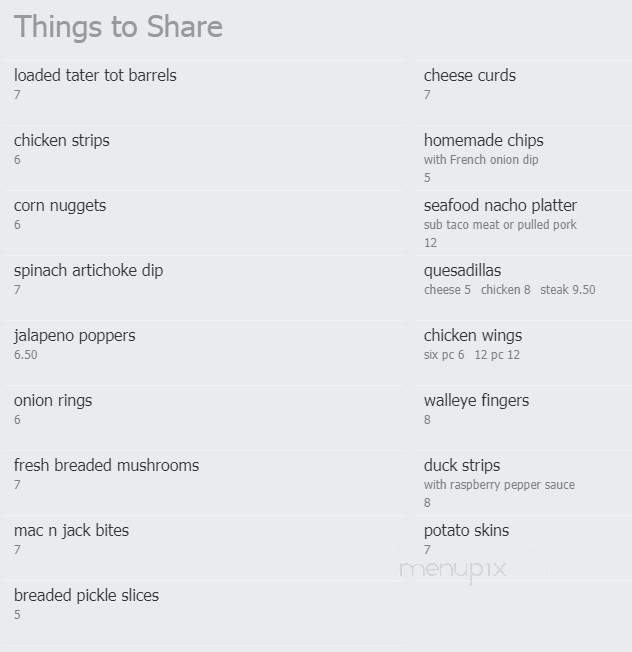*Screenshot of an Online Menu - "Things to Share" Section*

The image captures a portion of a digital menu on a light gray background, featuring a heading labeled "Things to Share" in the top left corner, distinguished by a darker gray backdrop. The menu items are meticulously organized into two columns with corresponding prices:

**Left Column:**
- Loaded Tater Tot Barrels - $7
- Chicken Strips - $6
- Corn Nuggets - $6
- Spinach Artichoke Dip - $7
- Jalapeño Poppers - $6.50
- Onion Rings - $6
- Fresh Breaded Mushrooms - $7
- Mac and Jack Bites - $7
- Breaded Pickle Slices - $5

**Right Column:**
- Cheese Curds - $7
- Homemade Chips with French Onion Dip - $5
- Seafood Nacho Platter (sub taco meat or pulled pork) - $12
- Quesadillas:
  - Cheese - $5
  - Chicken - $8
  - Steak - $9.50
- Chicken Wings:
  - 6 pieces - $6
  - 12 pieces - $12
- Walleye Fingers - $8
- Duck Strips with Raspberry Pepper Sauce - $8
- Potato Skins - $7

Below the list, the text "Menu Picks" is faintly visible in light gray. This screenshot effectively represents an "Online Menu" with listed items and prices available for sharing appetizers.